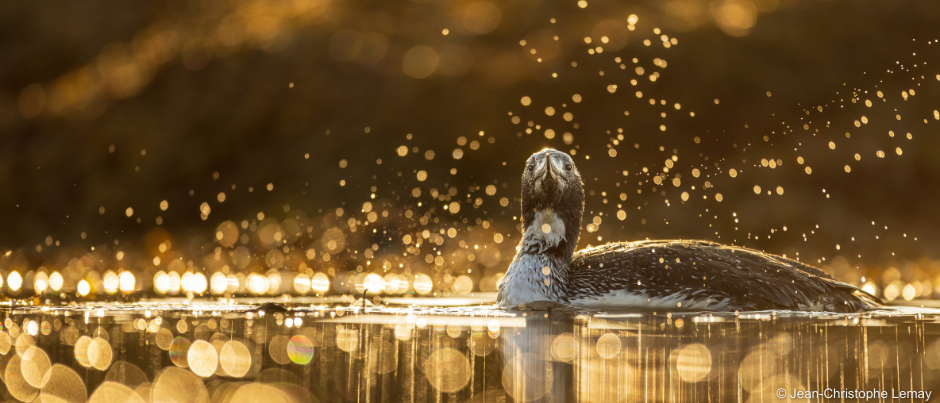The photograph is a stunning outdoor capture of a waterfowl, likely a mud hen, floating serenely on the surface of a lake. The rectangular, banner-shaped image showcases the bird half-submerged in the water, with its dark gray and brown feathers adorning its back and head, while its white neck and underbelly gracefully emerge from the golden water. The bird, looking straight at the camera with its yellow beak slightly pointed upwards, seems to be gazing inquisitively down its nose. The early daytime sun casts a yellowish-gold hue across the water, illuminating various golden spots from the splashes around the bird. Reflections shimmer off the surface, adding a magical quality to the scene. In the bottom right corner of the photograph, a white watermark reads "copyright, Jean-Christophe Lemay."